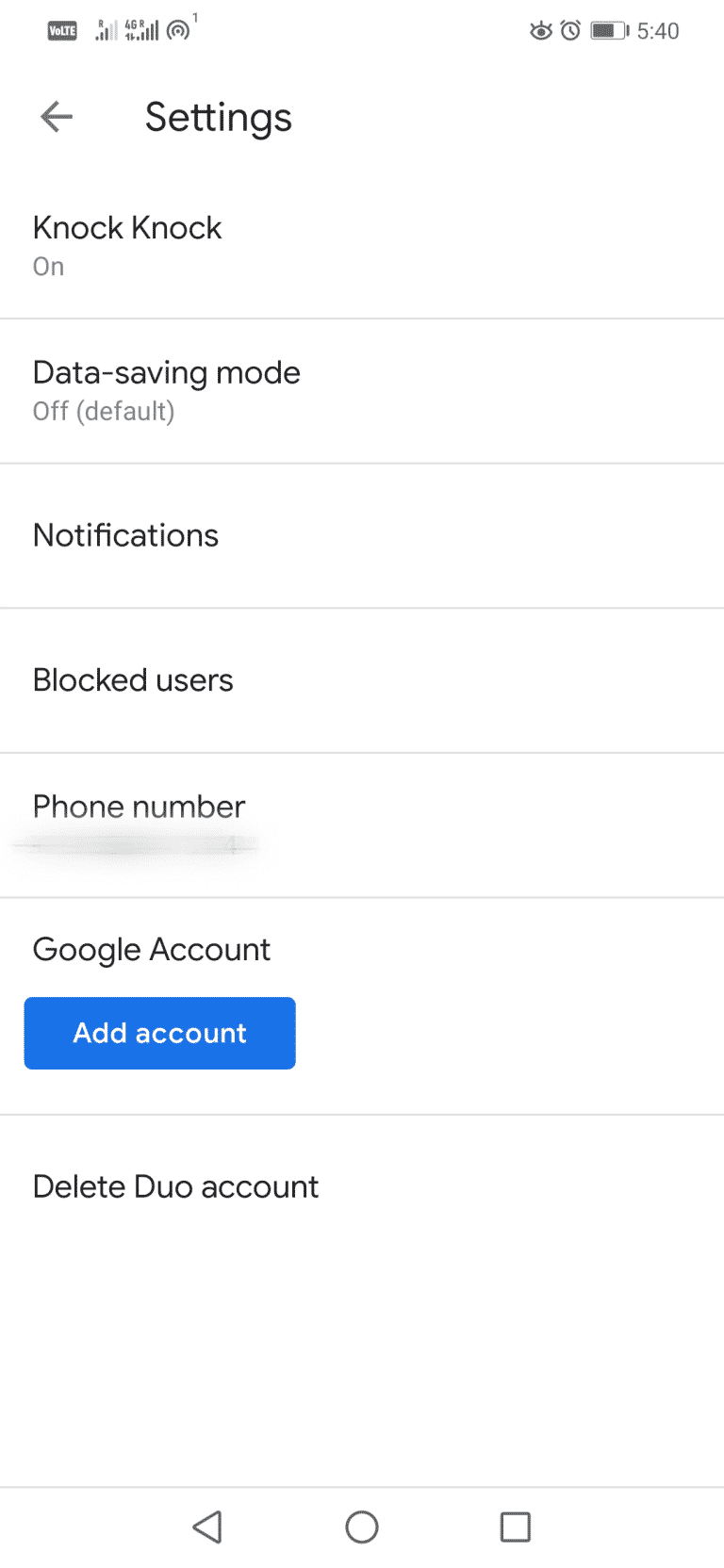A detailed screenshot from a phone depicting the "Settings" menu within an unnamed application. The image includes the following elements from top to bottom:

1. **Status Icons**: At the very top, in light gray, are tiny status icons. While hard to discern, an eye icon, a clock icon, a battery bar showing about three-quarters full, and the current time as "5:40" are visible.
  
2. **Navigation Header**: Below the status icons, there's a left-pointing arrow next to the word "Settings" in a larger font.

3. **Settings Options**: The settings options are divided by light gray horizontal lines:
  - **"Knock Knock" Option**: Listed as "Knock Knock" with the status "On."
  - **"Data-Saving Mode"**: Displayed as "Data-Saving Mode," marked "Off" with the note "(default)."
  - **"Notifications"**: Listed simply as "Notifications."
  - **"Blocked Users"**: Labeled as "Blocked Users."
  - *Blurred Section*: Under "Phone number," some information is deliberately blurred out.
  - **"Google Account"**: Listed as "Google account."
  - **Add Account Button**: A prominent blue rectangle with white lettering that reads "Add account."

4. **Final Option**: The last option reads "Delete Duo account."

5. **Navigation Bar**: At the bottom, there is a navigation bar containing three symbols: a triangle pointing up and to the right, a circle in the middle, and a rectangle all the way to the right.

Each section is separated by distinguishable, light gray lines, organizing the settings options clearly. The structured layout and easily navigable interface suggest an organized approach to managing app settings.